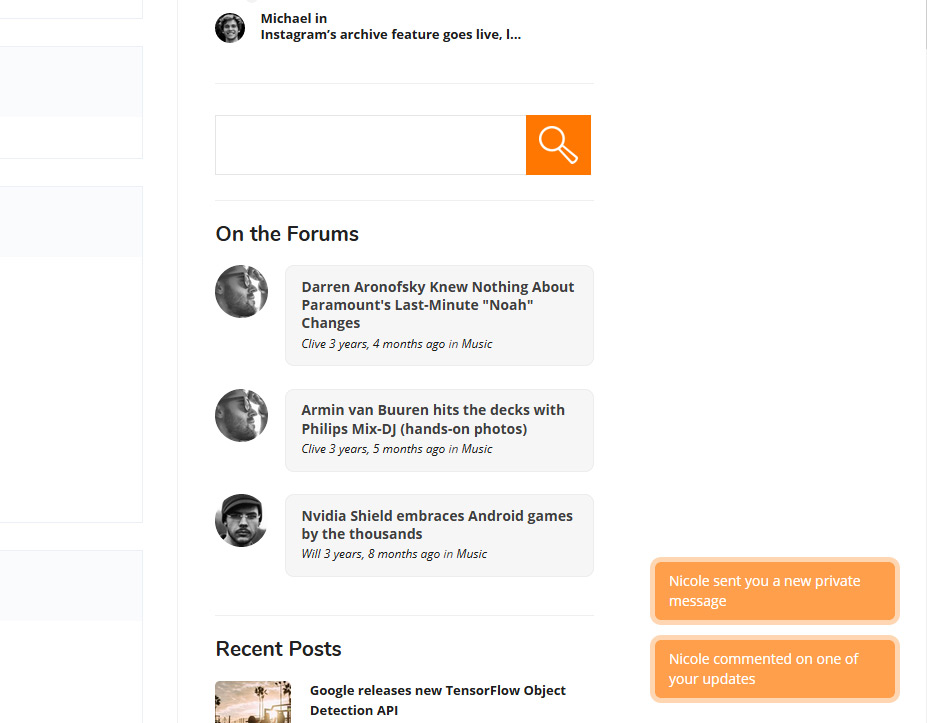The image features a social media post set against a white background. In the upper left, there is a man's face with the name "Michael" to the right, and the text "Instagram archive feature goes live." Below this is a white search box, and beneath the search box, in bold black text, reads a forum post titled "Darren Aronofsky knew nothing about Paramount's last-minute Noah changes," accompanied by the details "Clive, three years, four months ago." Below in the "Music" category is another post titled "Armin van Buuren hits the decks with Philips mix DJ hands-on photos" by Clive, from three years, five months ago. Further down is a black-and-white photo of a fair-skinned man with a beard, mustache, and a cap, with the caption "NVIDIA Shield embraces Android games by the thousands," posted by Will, three years and eight months ago, also in the Music category. On the right side, there are two orange notification boxes; the top one reads "Nicole sent you a new private message," and the one below it states "Nicole commented on one of your updates."